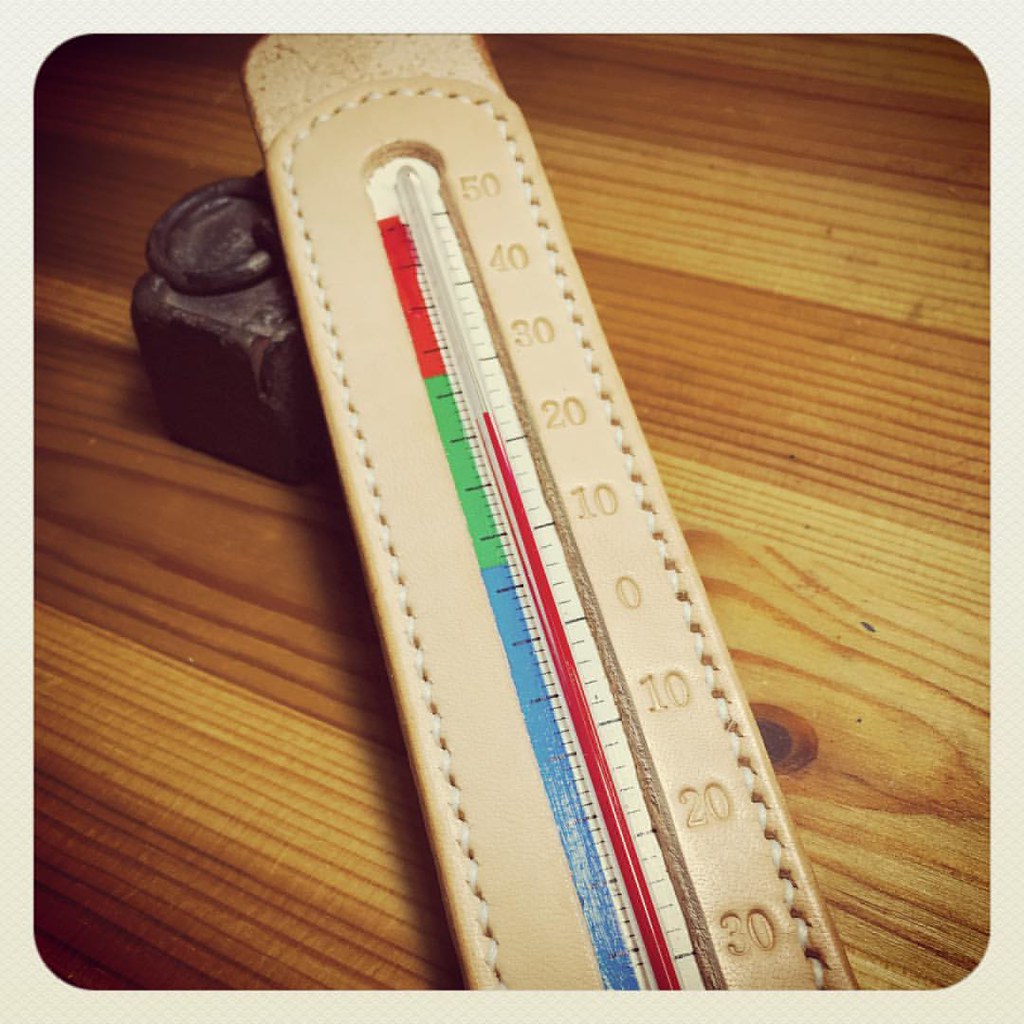This close-up photograph captures a vintage thermometer resting on a wooden desk, showcasing intricate details and textures. The thermometer, prominently positioned at a slight angle, features a white leather casing, meticulously stitched along its edges. Its central element—an elongated glass tube—displays a colorful gradient of red, green, and blue, visually charting temperature readings. Engraved directly into the leather are numeric indicators ranging from -30 to 50, prominently framing the temperature gauge. In the upper left corner of the image, a brown leather block adorned with a matching ring adds a rustic touch. The desk itself, with its rich wood grain displaying a spectrum from light to medium-dark brown, provides a warm and complementary background to the elegantly crafted thermometer.